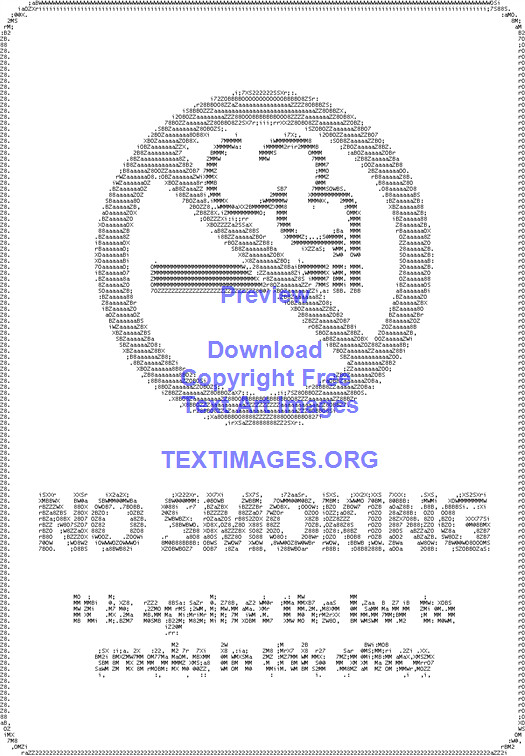The image is a vertical rectangular sign with rounded corners, featuring intricate, pixelated text and borders that appear to be made up of very small letters or numbers. At the upper middle part of the sign, there is a prominent "no smoking" symbol consisting of a cigarette with smoke, crossed out by a line from the top left to the bottom right within a circle. Beneath this circle, in blue letters, it reads: "preview," followed by "download," "copyright-free," and "text art images" arranged below each other. Lower down, it says "textimages.org" in blue letters. Continuing down the sign, in a pixelated font, large capital letters declare "NO SMOKING." Below this, it states, "It is against the law to smoke in the office." The border around the image is a thin line, also pixelated, contributing to the overall detailed, text-based design.